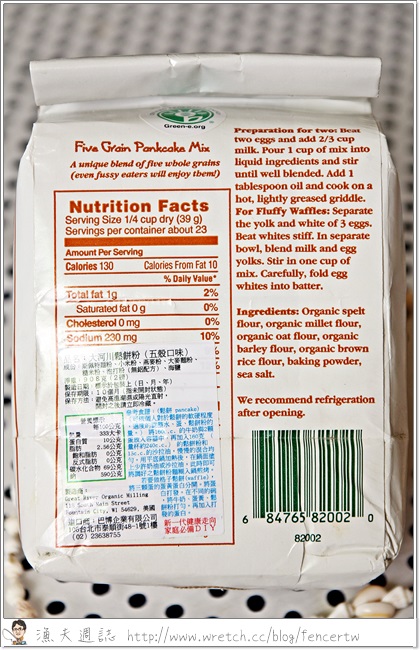This detailed photograph showcases the back of a product packet set against a surface with a white background adorned with black polka dots. A white strip runs along the bottom edge of the image, featuring a website address in gray text, hinting that this image may have been sourced from an online search. 

The product in question is a white bag, reminiscent of a flour bag, labeled as "Five Grain Pancake Mix." While the specific brand is not visible, the packet includes pertinent nutritional information written in English. Additionally, there is text in an oriental language, adding an international element to this product. 

On the right-hand side column of the packet, preparation instructions and a list of ingredients are provided, ensuring the user can easily follow the steps needed to create delicious pancakes. To complete the back label design, a barcode is positioned in the bottom left corner of the packet.